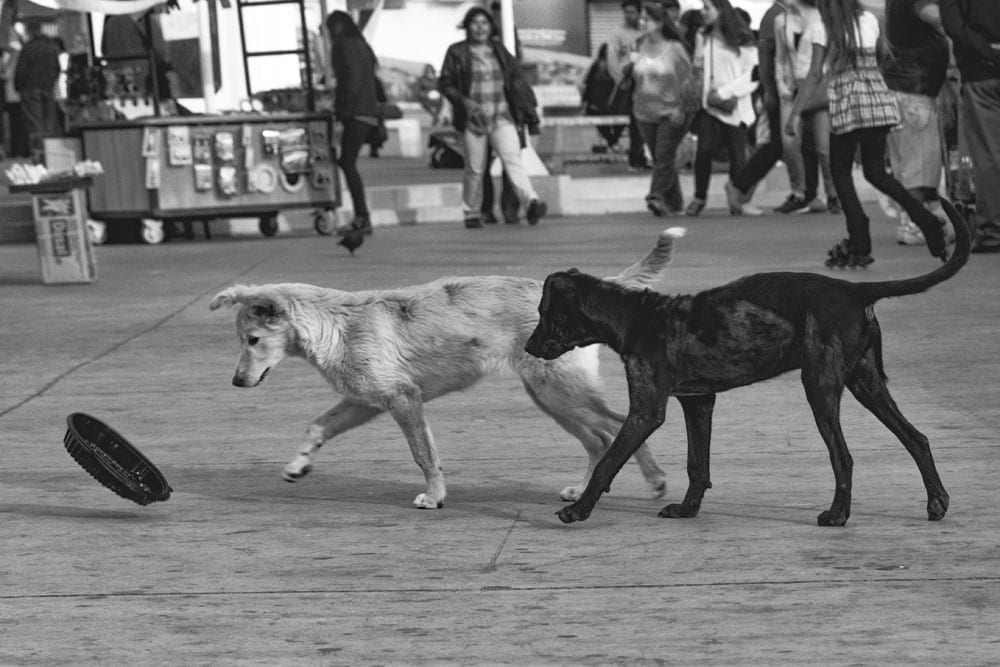This black and white photograph captures a vivid street scene featuring two dogs, one with light fur and the other with dark fur, seemingly of different breeds and without collars, chasing after a black disc. The action unfolds on what appears to be a bustling street, possibly part of a street fair or market. In the background, a diverse crowd of people can be seen moving in various directions, with several individuals' faces clearly visible. One notable figure is a girl with long hair, dressed in black tights and a skirt, who stands out on rollerblades. To the upper left, a vending cart or stand is present, partially obscured but attended by an individual in a black outfit. The overall lively atmosphere suggests a vibrant, outdoor setting, filled with shoppers, tourists, and vendors.